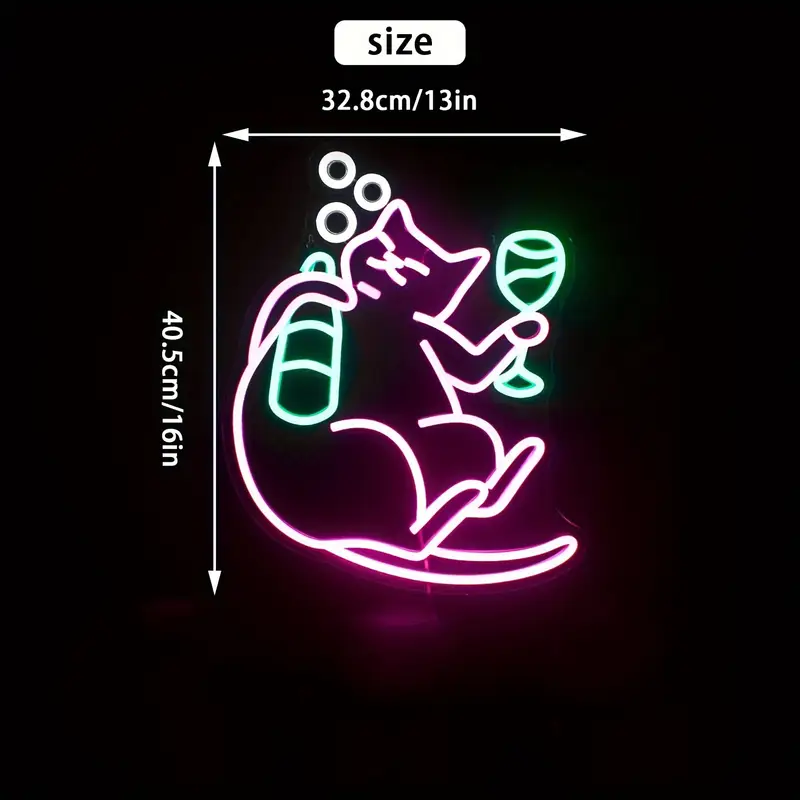The image depicts a digital neon sign against a black background, emphasizing the glow of the neon lights. The neon artwork features a playful scene of a cat, outlined in pink neon, reclining with its belly facing the viewer. The cat has pointed ears, visible eyes, and whiskers, and appears to be enjoying a drink with a green beer bottle in its left paw and a wine glass in its right paw. White bubble-like circles emanate from the beer bottle, adding to the sense of inebriation. The cat's tail curls underneath its plump body. Surrounding the cat are various measurement lines indicating dimensions in both centimeters and inches. Specifically, a white rectangle at the top of the image reads "size," followed by the measurements "32.8 centimeters / 13 inches." Horizontal and vertical arrows stretch across the cat, displaying these dimensions. This digital creation might be intended for signage or other material requiring precise sizing, and there's a touch of red in the design, enhancing the vibrancy of the neon aesthetic.